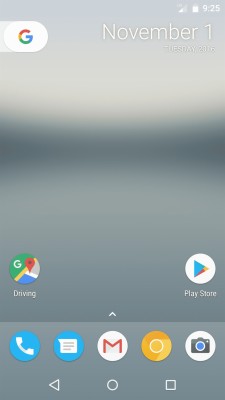The image is a screenshot likely taken from a tablet, set against a very blurry abstract background with hues of ivory, dark gray, and light gray. In the upper left corner of the screen, there is a toggle switch featuring the "G" from Google in its traditional rainbow array of colors. The toggle itself is white. In the upper right corner, icons display battery life, network reception, and the time, which reads 9:25. Directly beneath this information, the large white text shows the date as "November 1st, Tuesday 2016."

On the lower left of the screen, there is an icon for Google Maps labeled "Driving." To the right of this icon, there is a round white circle containing the triangular Google Play icon. The footer, depicted in a lighter gray, contains several icons: a white phone in a blue circle, a white message bubble in a blue circle, a red "M" in a white circle representing email, and a camera icon.